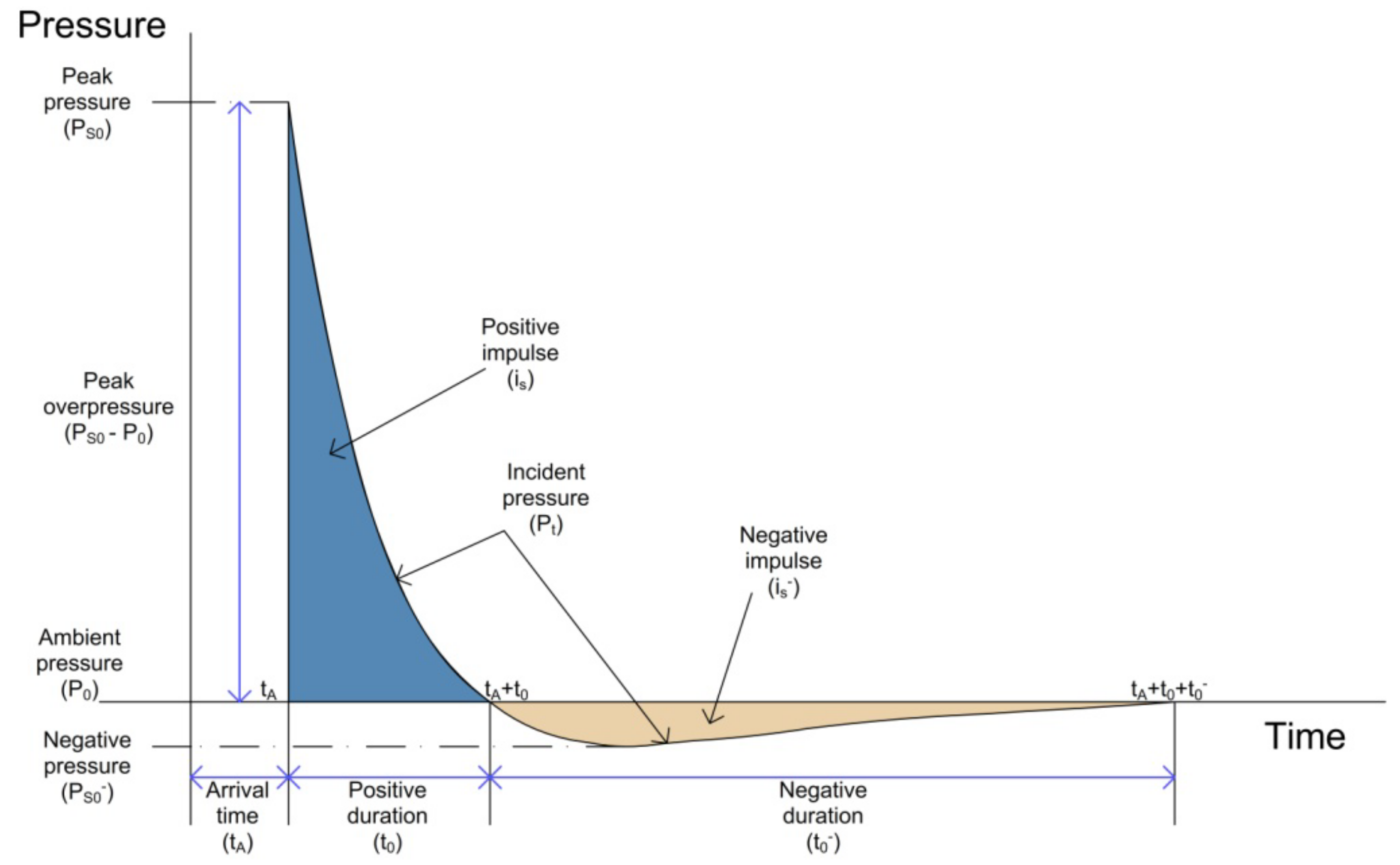This image features a detailed two-axis graph illustrating the relationship between pressure and time on a white background. The vertical axis (y-axis) is labeled "Pressure" at the top left in black font and includes the following sequence from top to bottom: Peak Pressure (PS0), Peak Overpressure (PS0 - P0), Ambient Pressure (P0), and Negative Pressure (PS0). The horizontal axis (x-axis) is labeled "Time" and lists Arrival Time (TA), Positive Duration (T0), and Negative Duration (T0). 

Within the chart, two different colored areas depict distinct aspects of impulse: the blue area represents Positive Impulse (IS), and the tan area signifies Negative Impulse (IS). The chart features black arrows and additional labels to enhance clarity: a black arrow points towards the blue area labeled as "Positive Impulse," another arrow points towards both blue and tan areas labeled as "Incident Pressure" (PT), and a final arrow directs towards the tan area labeled as "Negative Impulse." Overall, this graph effectively conveys the variations in pressure over time, highlighting both positive and negative impulses through its use of color and comprehensive labeling.